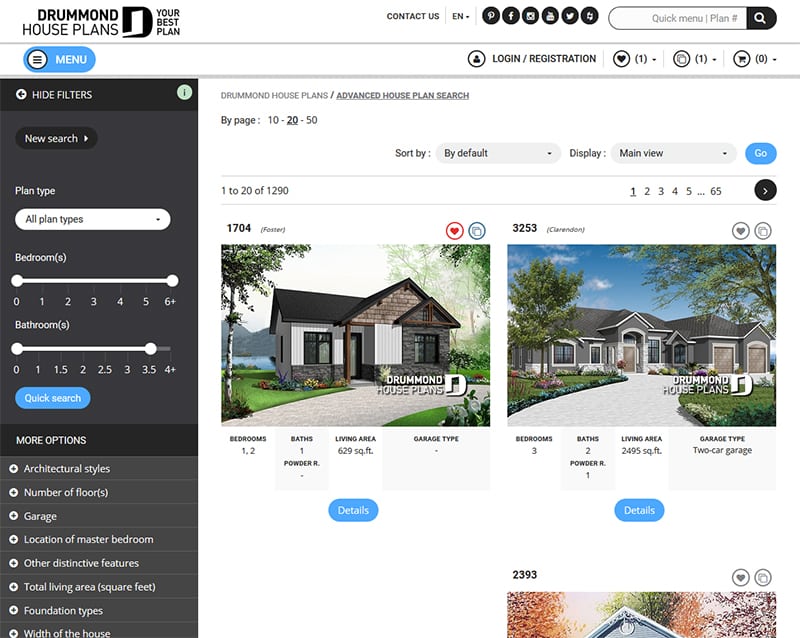The image displays a user interface from the Drummond House Plans website. The upper section against a white background features text in black reading "Drummond House Plans, Your Best Plan," followed by "Contact Us" and "English." Next to this text are buttons for social media platforms: Pinterest, Facebook, Instagram, an unclear icon, and Twitter. 

Below these top elements, there is a quick menu search bar. On the left, a blue button labeled "Menu" is prominently placed, while to the right are black text links for "Login" and "Registration."

On the left sidebar, a black column features white text for various filters, stating "Hide Filters," "New Search," and "Plan Type." Users can select from "All Plan Types." Below, there are sliding scales for selecting the number of bedrooms (ranging from 0 to 6+) and bathrooms (from 0 to 4+). A blue "Quick Search" button is situated underneath these filters. Additional options provided include "More Options," "Architectural Styles," "Number of Floors," "Garage," "Location of Master Bedroom," "Other Distinctive Features," "Total Living Area," "Square Feet," "Foundation Types," and "Width of the Home."

On the right, the main content area with a white background displays prominently. At the top, black text reads "Drummond House Plans Advanced House Plan Search." There are pagination options for displaying 10, 20 (selected), or 50 items per page. The interface includes an area for sorting and displaying results. Below this, there are two color photographs showcasing the exteriors of different homes, each accompanied by details and blue buttons labeled "Details."